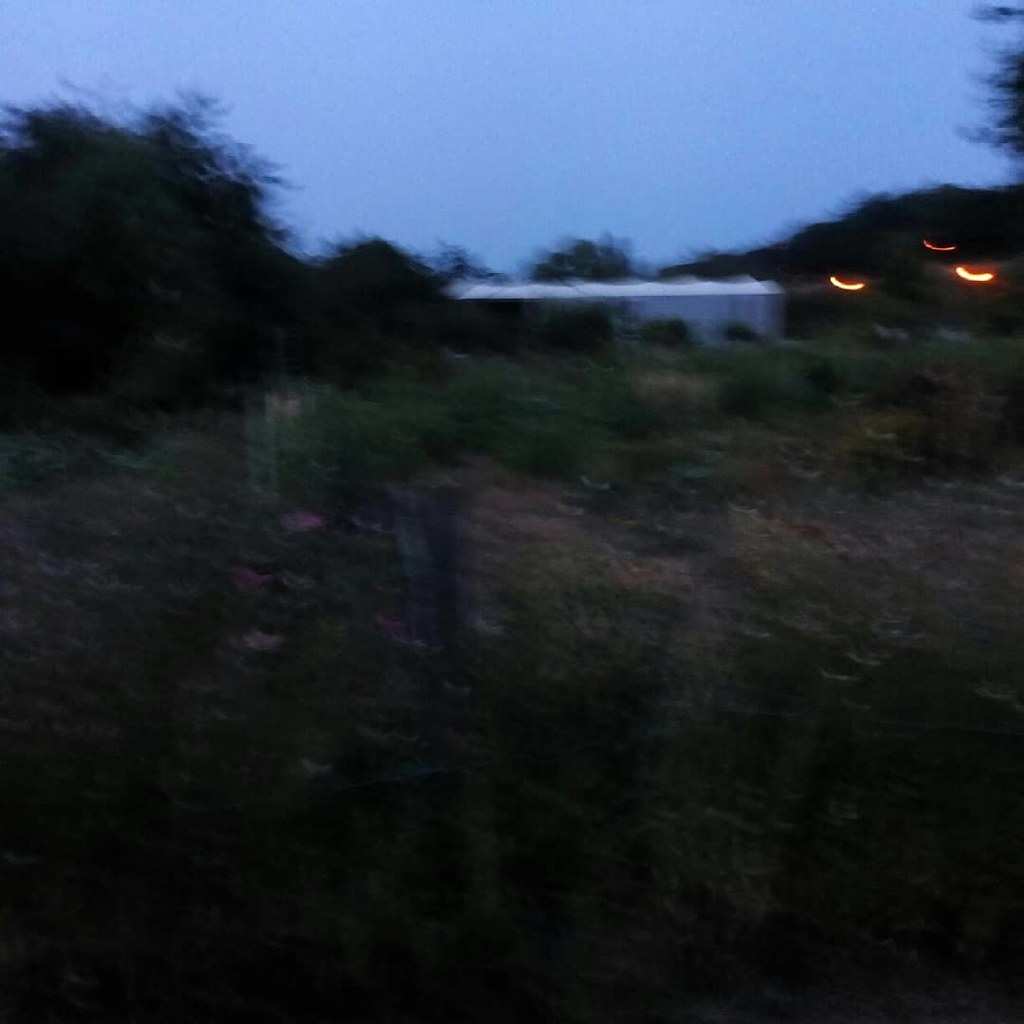Here is the cleaned-up and formulated detailed caption:

The blurry photograph captures a grassy field at dusk, with the tall grass predominantly green but transitioning to brown in spots on the right. There is a scattering of bushy trees lining both the left and far right sides. Dominating the center of the image is a metal shack-like structure. Off to its right is the faint silhouette of a hill, which stands out due to three bright, orange, cheeto-shaped lights glowing in front of it. The dark gray sky adds to the dim atmosphere, accentuating the shadows and dim flashes of color. The poorly focused image suggests a mysterious outdoor scene with both natural and man-made elements, woven together under the fading light of dusk.